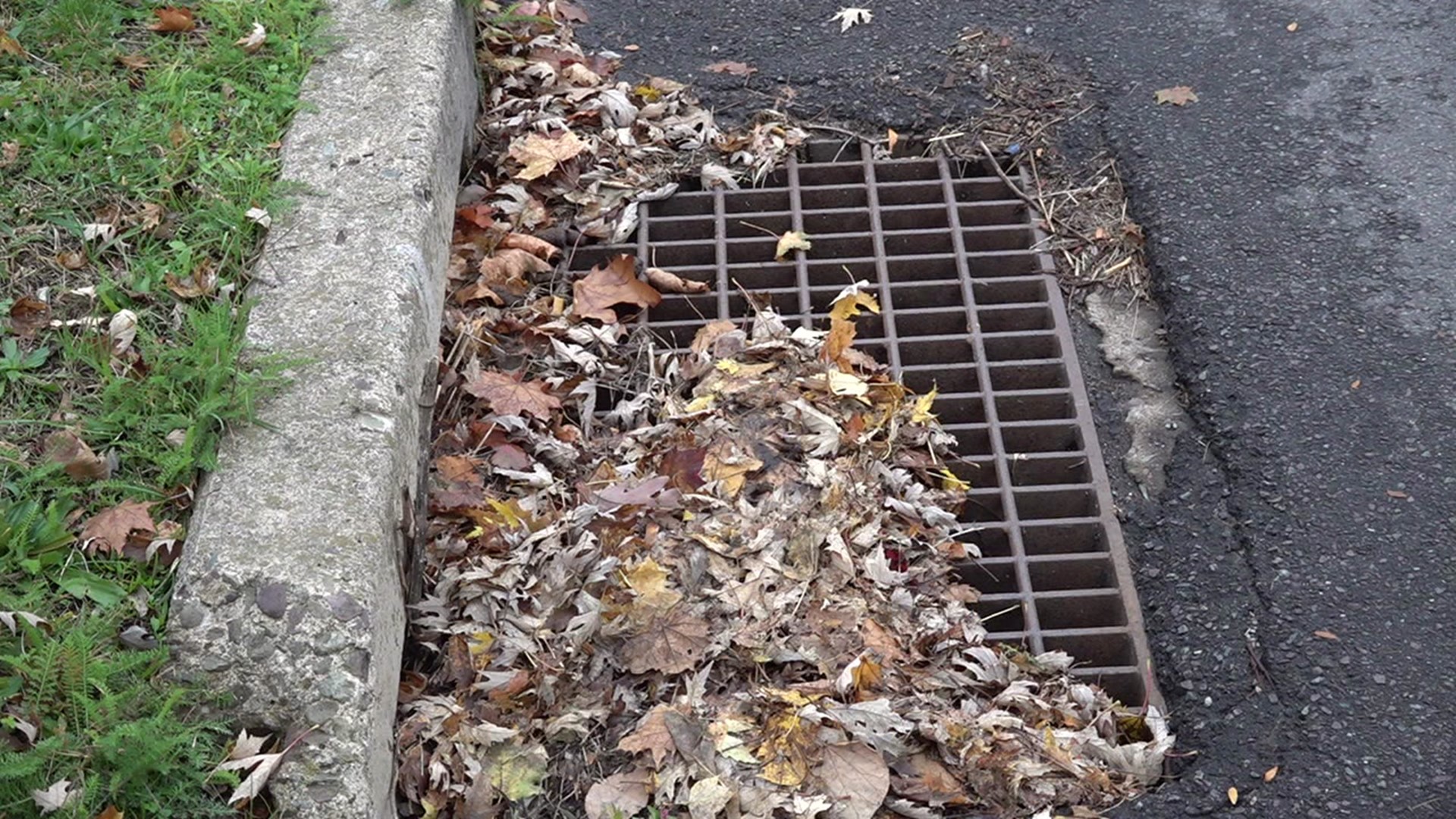This color photograph, taken in landscape orientation, captures a detailed view of a suburban drainage area on a paved street. Centered in the image is a metal drain grate, positioned vertically like a rectangle, partially clogged with a thick layer of autumn leaves and other debris. The grate starts at the bottom of the image and extends slightly towards the top, covered in places by a mix of wet, darkened leaves that form a diagonal blockage from the top left to the bottom right. To the left of the grate, a concrete curb runs parallel, leading up to an overgrown lawn with visible weeds and vegetation. The curb appears broken near the bottom edge of the image. On the right side, a black, wet tar road completes the scene, emphasizing the contrast between the materials and the autumn setting. The overall colors—shades of green, gray, black, brown, orange, and white—reflect the season's palette, framing a typical suburban street scene on an overcast day.